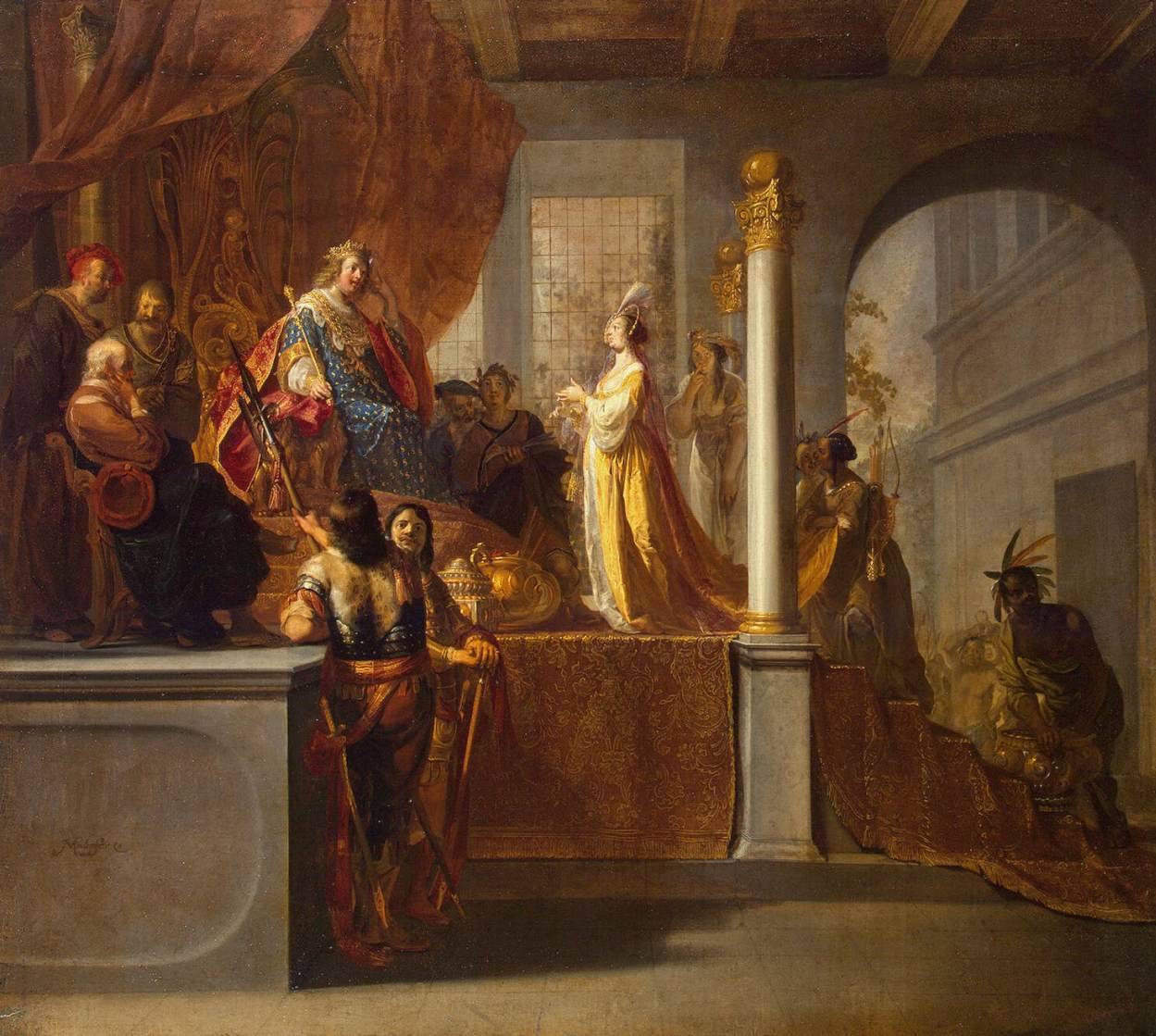The painting, reminiscent of Renaissance art, depicts an opulent scene set in a grand castle room adorned with massive pillars and huge doorways. At the center, on a pedestal resembling a stage, sits a king dressed regally in a long, royal blue robe with a red cape and a golden crown atop his head, accentuating his ginger hair. The king is either engaged in conversation or attentively listening to a woman who approaches him, standing at the forefront of the painting. The woman is elegantly dressed in a long gold gown with white sleeves and wears a distinctive headpiece adorned with feathers.

Surrounding them, the setting is vibrant with other figures. Seen on the steps leading to the king’s throne are various attendees, including advisors and courtiers. Of notable mention is a man, possibly of Indian descent, characterized by a feathered headdress, leaning over and engaging with the scene. Behind the king, two individuals can be seen, one appearing to hold a musical instrument like a lute or a bag. There are also men standing beside the stage, holding large swords aloft, adding to the solemnity of the atmosphere.

The color palette of the painting is rich and vivid, with predominant shades of gold, red, burgundy, and blue set against the gray stone walls of the castle. In the background, through the large window openings, a glimpse of the outside world is visible, showcasing lush green trees and foliage, adding a serene touch to the otherwise formal setting. The intricate details and historical attire suggest the painting would be a fitting exhibit in a prestigious museum like the Getty Center.